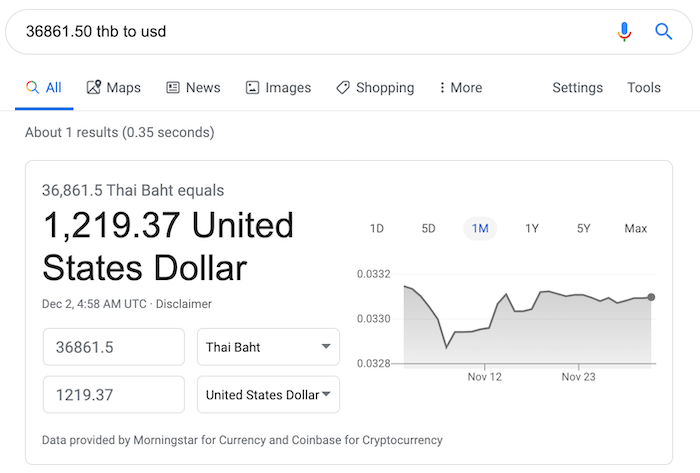A screenshot of a Google search conducted on a computer or laptop in landscape mode. The user searched for "36,861.50 Thai bahts" to find its equivalent in US dollars. The top of the screen displays the original search query, and below it, the interface offers options to navigate through various types of search results, including All, Maps, News, Images, Shopping, and More, with Settings and Tools on the far right. The search results show that 36,861.50 Thai bahts is equal to $1,219.37 USD, with the information processed in 0.35 seconds. A small chart on the screen indicates that the data is provided by Morningstar for currency and Coinbase for cryptocurrency. The background of the screenshot is predominantly white, featuring blue and black text.